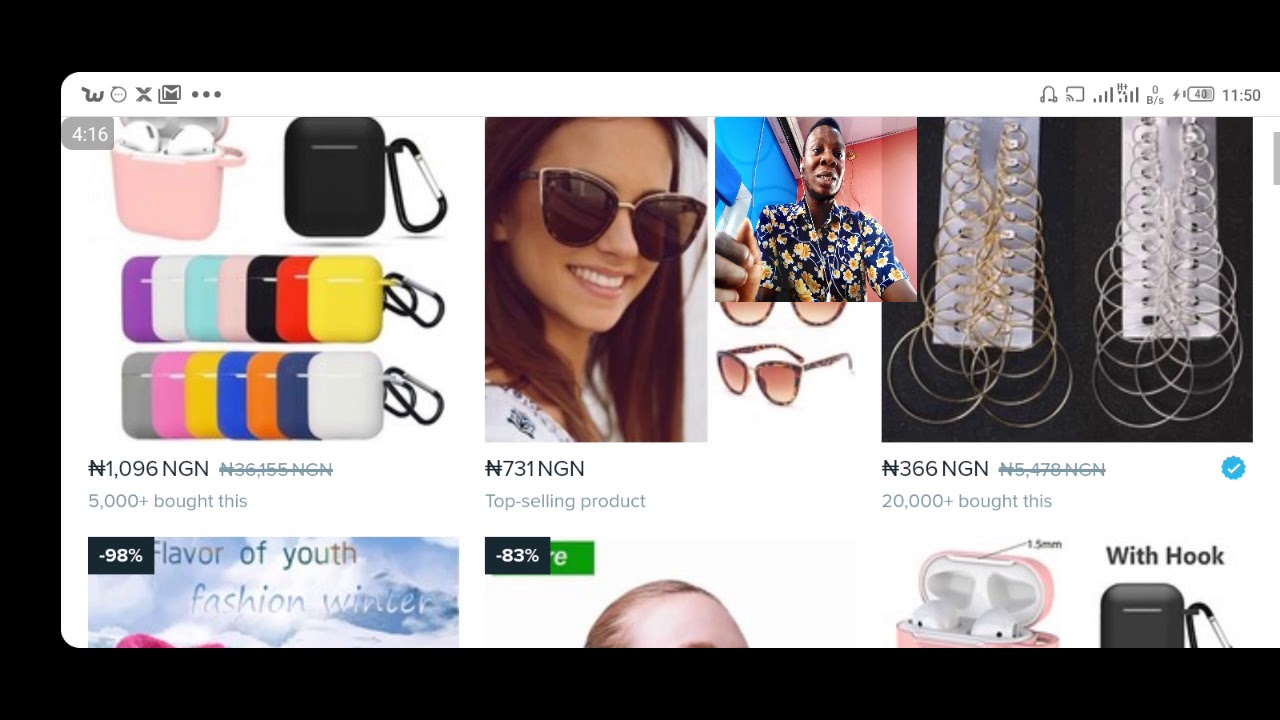The image appears to be a chic promotional display from a shopping website, likely viewed on a mobile device as indicated by the headphone icon and cellular signal in the upper right corner. On the left side, there are icons including a 'W', an 'X', an envelope, and three dots, with the time "4:16" displayed above. The main content showcases popular items purchased by many users, with a banner stating that 5,000 people bought a particular item. Featured products include stylish AirPod holders, modeled by a young Caucasian woman wearing oversized brown sunglasses, and an African-American man in a vibrant blue and yellow shirt. Additionally, there is a display of gold and silver loop earrings against a white background. At the bottom of the screen, it notes that 98% of viewers also considered other products, highlighting user engagement with the featured AirPod holders.